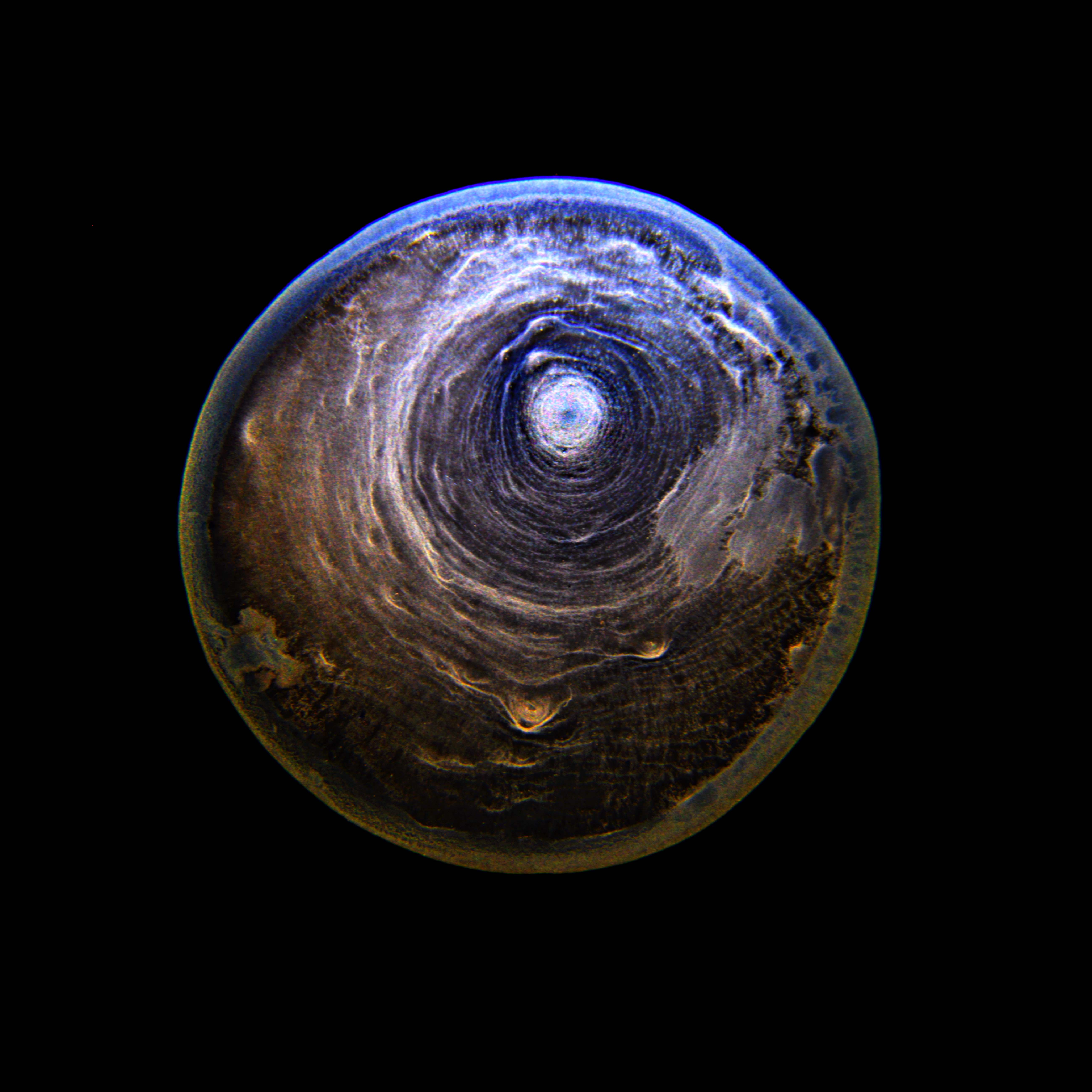The photograph showcases a captivating, circular orb set against a stark black background, exuding an aura of mystery and artistry. The orb's intricate design features a spectrum of colors and textures. The upper portion is bathed in blue hues, gradually transitioning to darker shades of green as it extends downward. The surface is interwoven with various swirls and textures, creating an effect reminiscent of circles within circles, or the view down a tube. The center is especially striking, with a defined swirl pattern that echoes the blue and purplish tones found at the top. The orb's design suggests it could be an abstract piece of art or a detailed model, possibly a beautifully painted object or perhaps a blown glass formation. The light plays a significant role, highlighting the orb's top section and casting subtle gradients that add to the overall depth and dimension of the piece, making it resemble everything from a planet to a stylized eyeball.